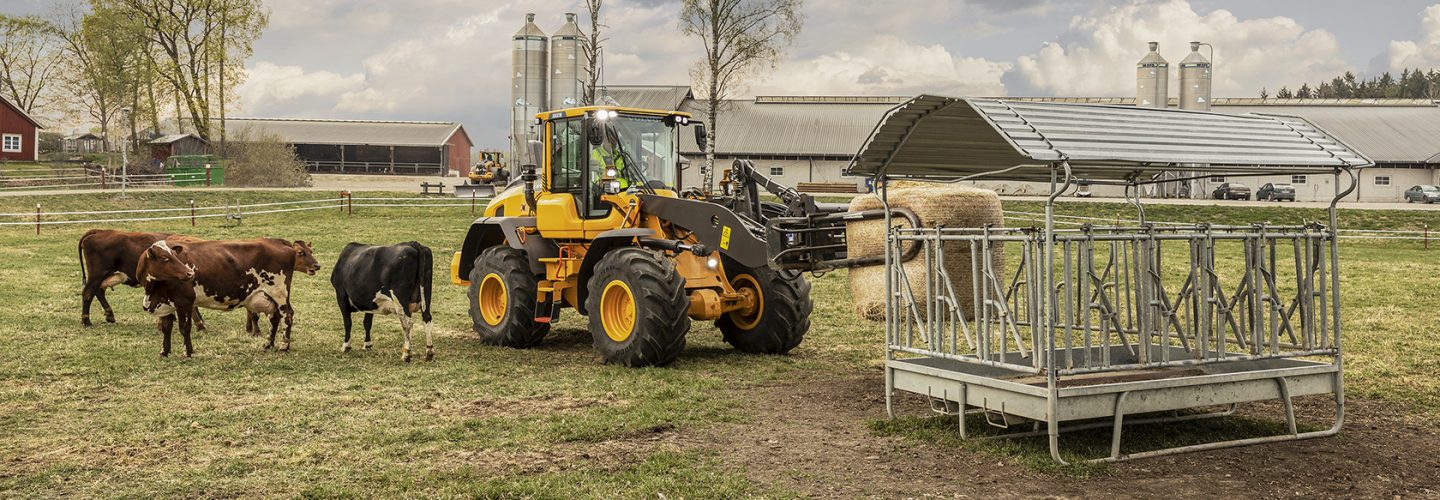In the photograph, there is a wide-angle view of a dairy farm under a gray, cloudy sky. Prominently featured is a yellow Caterpillar-like tractor with large black wheels, using its front clamp to hold a sizeable square hay bale. Nearby, the tractor is positioned near a metal trough with an overhang, possibly used for feeding or washing the cows. To the left of the tractor stand four cows: three are brown with white spots, and one is black with white markings.

In the background, lush green grass and patches of dirt define the landscape, which is encircled by what appears to be an electrified fence. Set against a backdrop of tall trees with green leaves, there are several farm buildings. A red structure with a white-framed window stands out, along with a distant brick building featuring a gray roof. This expansive scene captures the essence of life on a functional dairy farm.